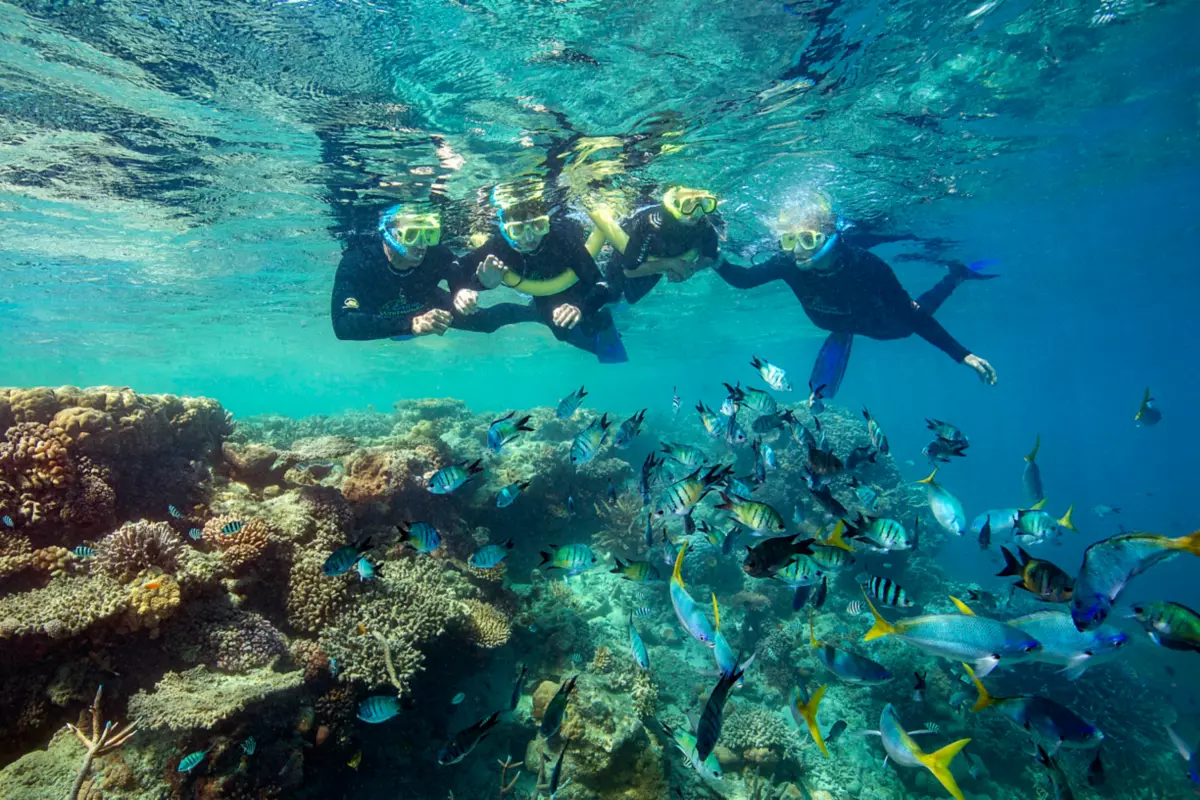This underwater image captures an enchanting marine scene where four scuba divers, donned in black wetsuits and yellow goggles, are suspended just below the water's surface. Their heads likely emerge from the greenish-blue, hazy water, the overall effect enhanced by the blue-tipped snorkels and flippers. Two divers hold long, tubular floats against their stomachs. Beneath their wading forms, the vibrant marine life flourishes. Various colorful fish, predominantly turquoise with yellow tails and some with distinctive black stripes, swim lazily around an array of corals. These corals exhibit shades of beige, purple, and orange, accented by additional marine flora. Concentrated toward the bottom right of the frame, the marine display adds a vivid burst of life to this serene underwater tableau.